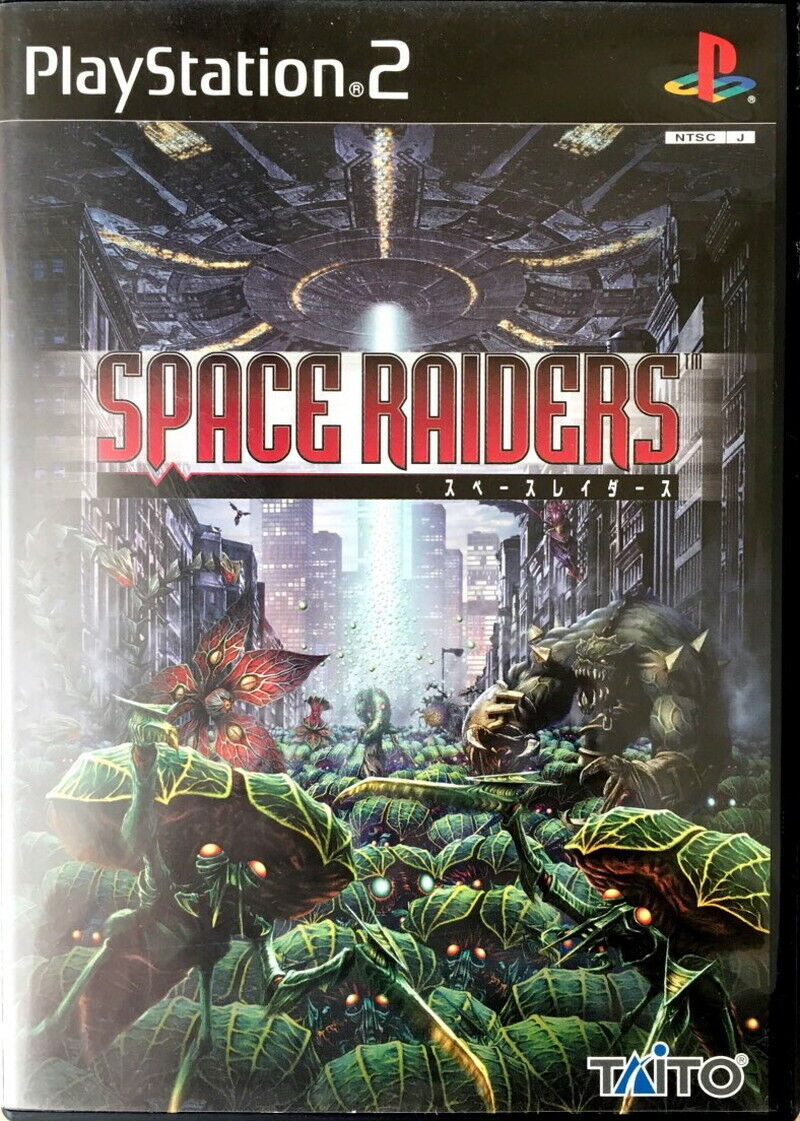The PlayStation 2 game cover for "Space Raiders" prominently displays its title in stylized red, all-caps font across the middle with a black rectangle beneath it, containing white Japanese text. The PlayStation 2 branding is found at the top left in a white font on a black rectangular background, while the top right showcases the interlocking P (in red) and S (in yellow, green, and blue) PlayStation logo, accompanied by the NTSCJ designation. The bottom right corner features the Taito logo. The cover art itself illustrates an intense urban scene of skyscrapers under attack by various aliens, including towering green monsters and red flower-like creatures. A spaceship hovers above, casting a beam of light down onto the chaos below, enhancing the sense of an extraterrestrial invasion.